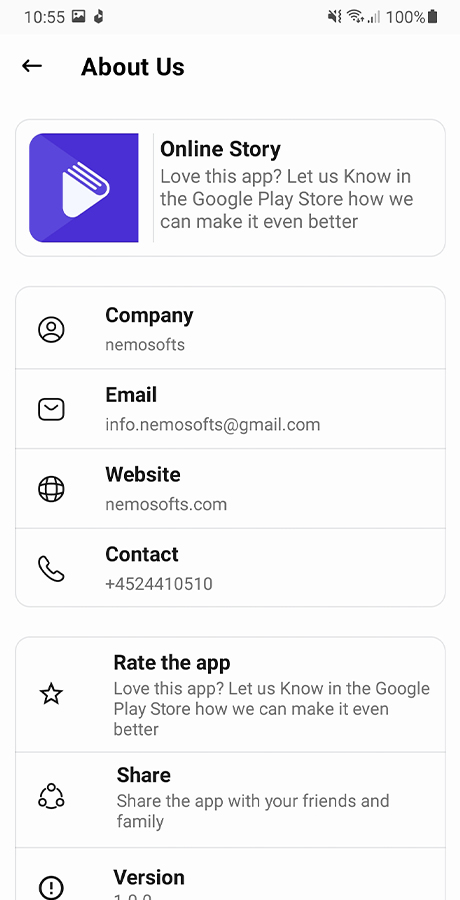The image is a screenshot of a smartphone displaying various app-related information and indicators. At the top, the status bar shows the current time, battery life, and WiFi signal strength. Beneath this, a navigation bar includes a back arrow and the text "About Us" in black. Further down, the text reads, "Online Story," followed by a promotional message: "Love this app? Let us know in the Google Play Store how we can make it even better."

A purple icon with a shining white light in the center is prominently featured. Below it lies a section labeled "Company: NemoSofts," which includes an outline of a person's head. The contact details for the company are listed:

- Email: info.nemosofts@gmail.com, accompanied by a white mail envelope icon.
- Website: NemoSofts.com, paired with a globe icon.
- Contact Number: 452-441-0510, indicated by a cell phone icon.

The "Rate the App" section reiterates the message of user feedback: "Love this app? Let us know in the Google Play Store how we can make it even better." The "Share" section invites users to share the app with their friends and family. Lastly, a "Version" section features an exclamation mark enclosed in a black circle and indicates that the app version is 1.00.